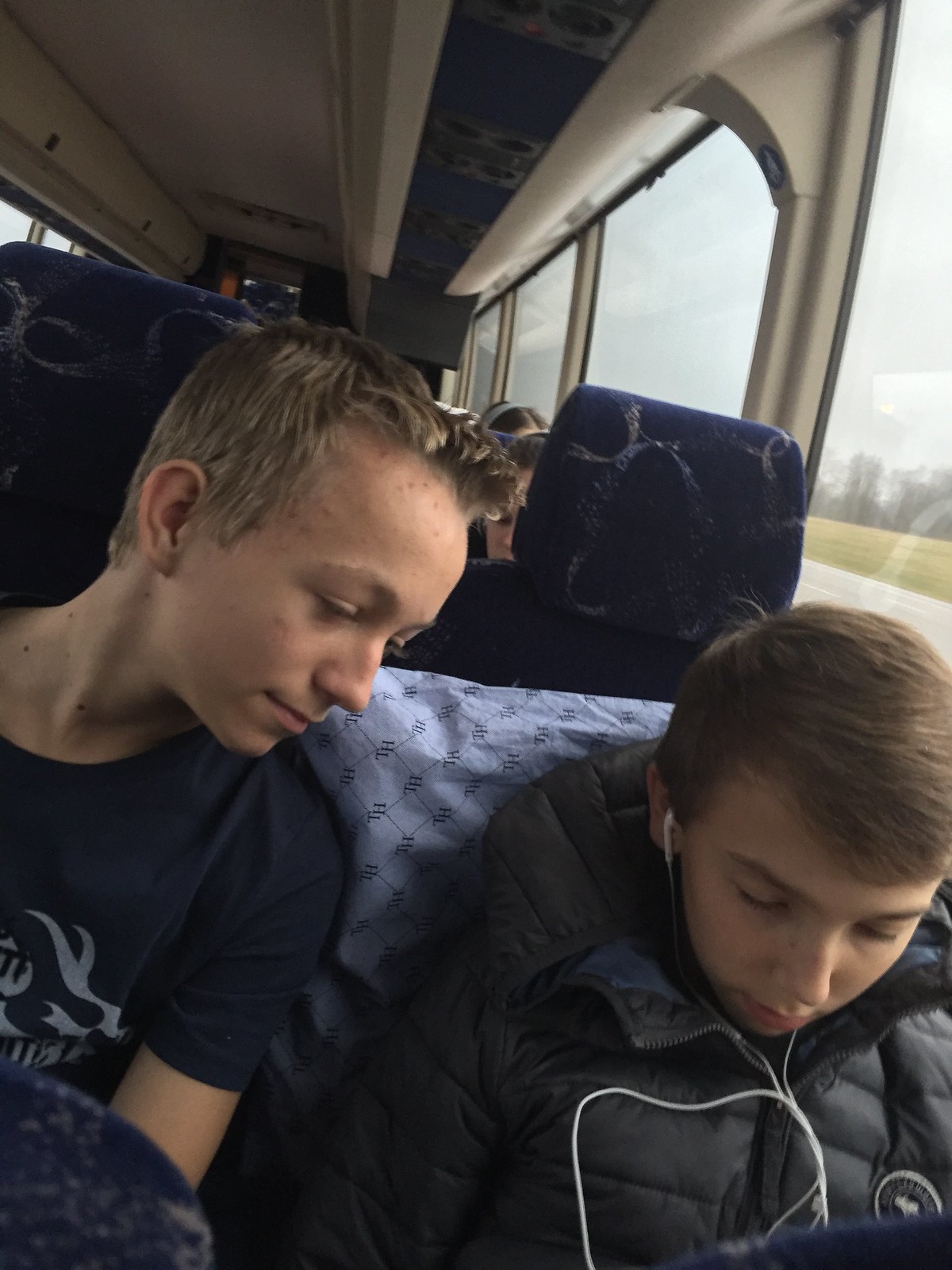The image depicts two younger individuals seated on what appears to be a bus, potentially a train, each in their own seats equipped with blue headrests. A light blue pillow is visible behind one of them. To the right is a boy wearing a dark puffy jacket, with corded earphones around his head, seemingly plugged into a device. He has brown hair and is looking down, likely at a phone or another electronic device. To his left, there is another boy with a shorter haircut and blonde hair, dressed in a dark t-shirt with a light-colored logo, also intently focused on the shared electronic device. Both seats they occupy are blue. In the background, large windows reveal a scenic countryside landscape featuring a line of trees, blue skies filled with clouds, a green field, and a street. This setting inside what seems to be a white bus suggests a journey through a rural area.